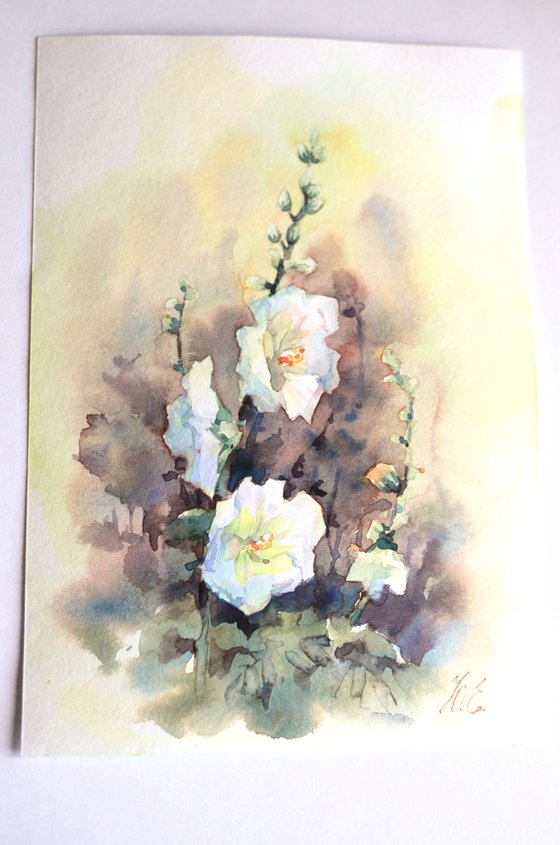This image is a detailed watercolor painting, set on a white surface. The composition features three prominent white flowers in full bloom at the center, with an additional smaller white flower to the right. Surrounding the main flowers are various buds in different stages of opening, with most remaining closed. The flower stems are painted green, blending seamlessly with green leaves that extend outwards towards the top and sides of the painting.

The background of the painting is a mixture of creamy white, dirty yellow, and brownish shades, with hints of purplish, grayish, and bluish tones interspersed throughout. The artist utilized black to depict shadows under the leaves and flowers, adding depth and contrast. This interplay of colors makes the white flowers stand out prominently against the varied background. The painting also includes the artist's signature located on the bottom right-hand corner. Despite not being exceptionally clean, the use of mixed colors and deliberate brush strokes highlight the artist's unique style, contributing to the overall aesthetic appeal of the artwork.